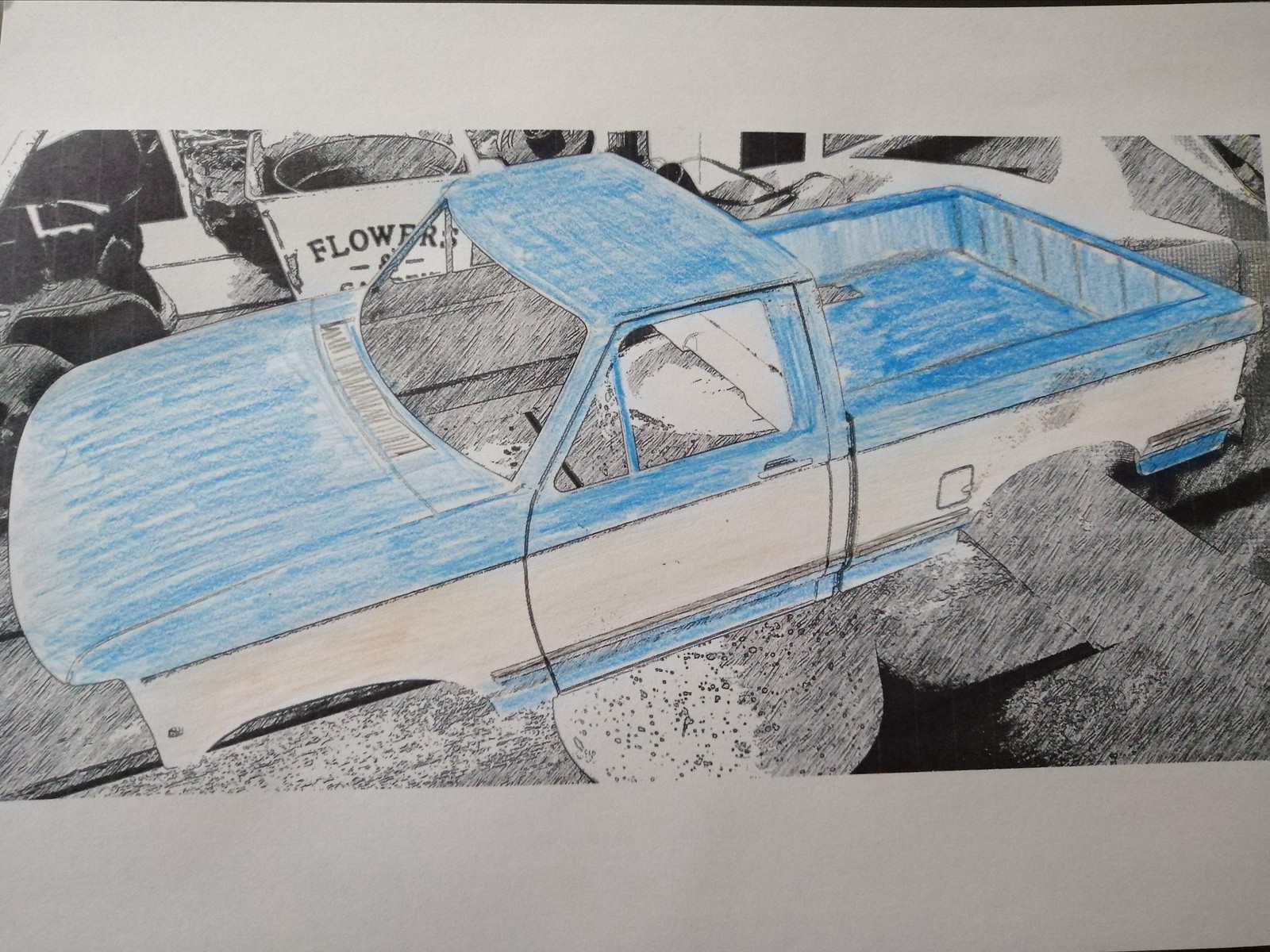This hand-drawn image depicts a blue pickup truck, meticulously sketched with a pencil and colored in with blue crayon, evident from the thick, slightly wavy lines. Central to the drawing, the truck is devoid of wheels and axles, appearing as just the bed and frame. The truck's body features a prominent, white stripe running horizontally from the front to the back, with blue extending above and below this line, complemented by black shading beneath it. The interior is visible but vacant, lacking seats and a steering wheel, giving a skeletal appearance. Additionally, a gas cap is drawn near the stripe. Positioned in what resembles a scrapyard, the truck is surrounded by incomplete vehicles amidst an unclear, grayish surface. Notably, to the left side of the truck, there's a partially visible container with the word “flowers” inscribed, indicating a backdrop filled with subtle yet significant details.